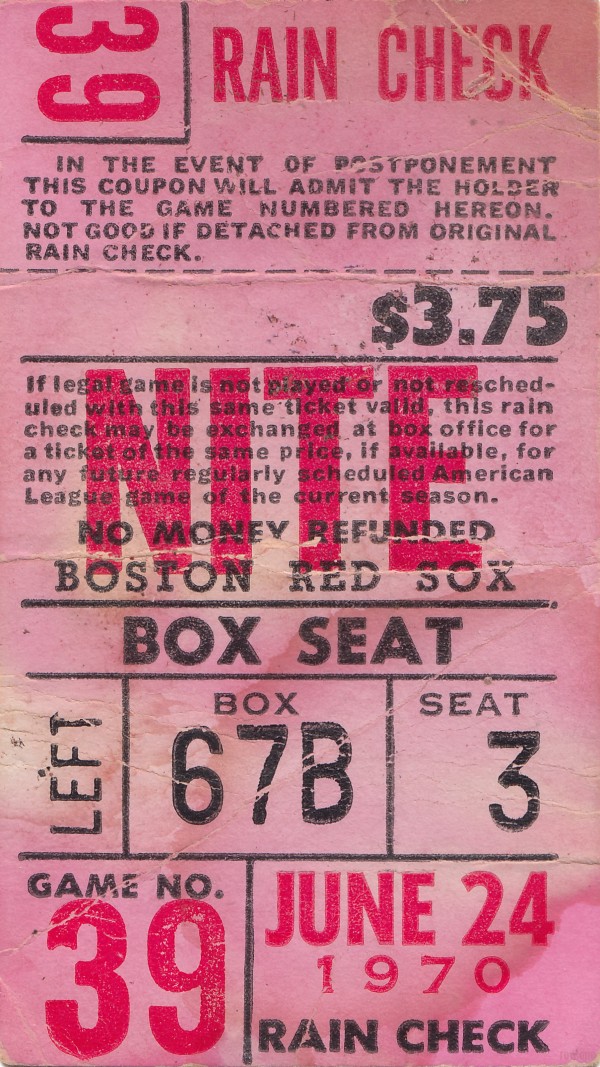This vintage Boston Red Sox ticket, dated June 24, 1970, is titled "Rain Check" in all capital letters at the top right, highlighted in hot pink. The number "39" appears prominently on the top left. Priced at $3.75, the ticket is for game number 39, valid for a box seat in section 67B, seat number 3, on the left side. A note below the "Rain Check" title in black text states: "In the event of postponement, this coupon will admit the holder to the game numbered hereon. Not good if detached from original Rain Check." Additionally, it mentions that if a legal game is not played or rescheduled, the Rain Check can be exchanged at the box office for a ticket of the same price, subject to availability, for any future regularly scheduled American League game of the current season. The bottom right corner also features "Rain Check" in bold, black capital letters.